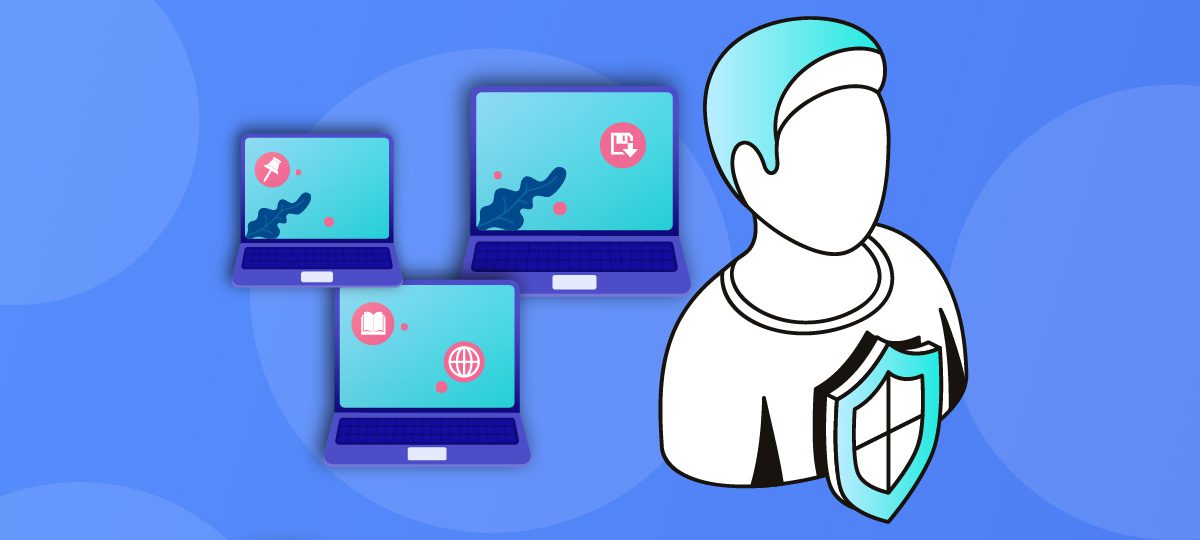The detailed horizontally-aligned rectangular animated graphic displays a vivid blue background adorned with patterns of large, subtly shaded circles in varying blue hues. Centrally and to the left side of the image, three slightly different-sized opened laptops are positioned vertically in a staggered arrangement. Each laptop screen showcases a green background with unique iconography: the top-left laptop features a leaf and a thumbtack, the top-right laptop displays a leaf, a disc, and an arrow encircled, while the bottom-center laptop shows two circular icons depicting a globe and an open book. The laptop keyboards are characterized by a purple hue with contrasting blue keys. To the right of the laptops, a silhouette of a person's upper body is illustrated, featuring a white circular face with a black outline, adorned with blue or green hair. The figure wears a white shirt and a green shield on their chest, enhancing the graphic's animated and cohesive design.